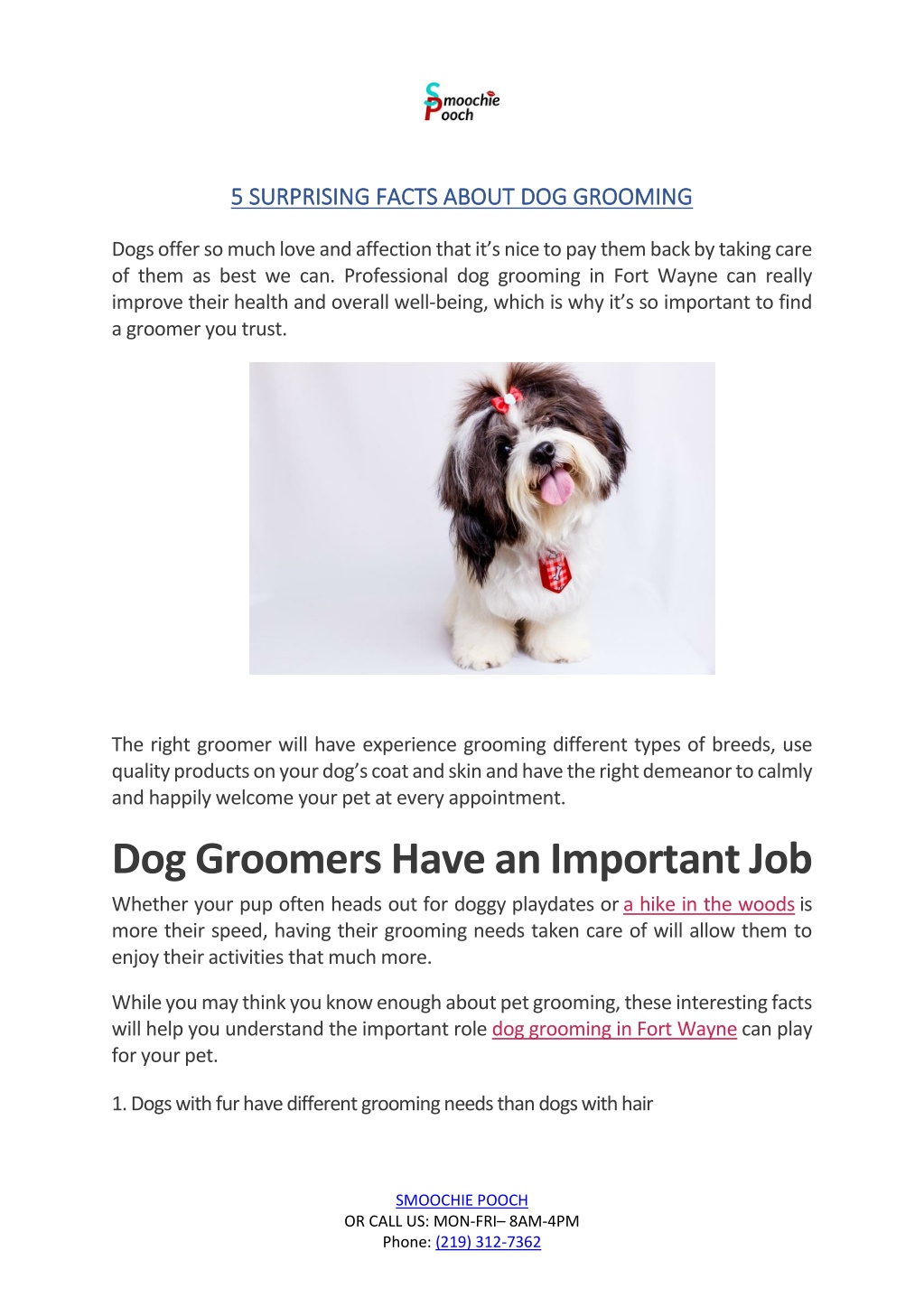**Caption:**

---

On a pristine white background, the focus is drawn to the center where the words "Smoochy Pooch" are creatively displayed, with the 'S' designed to resemble a playful tail and the 'P' colored in red. Below, a blue underline highlights the phrase "Five Surprising Facts About Dog Grooming." In smaller black text, a message conveys the deep affection dogs offer and the importance of reciprocating their love through proper care: "Dogs offer so much love and affection that it's nice to pay them back by taking care of them as best we can. Professional dog groomers in Fort Wayne can really improve their health and overall well-being, which is why it's so important to find a groomer you trust."

Beneath this text is an adorable photo of a small dog with a red bow on its head. The dog's fur is primarily white with patches of dark gray and white, and it wears a matching red and white collar. Just below the image, another informative message is presented, reinforcing the importance of choosing the right dog groomer: "The right dog groomer will have experience grooming different types of breeds, use quality products on your dog's coat and skin, and have the right demeanor to calmly and happily welcome your pet at every appointment."

Emphasized in bold, "Dog groomers have an important job," the text continues in regular font, mentioning various common activities for dogs: "Whether your pup prefers heads of doggie playmates or," in red and underlined, "a hike in the woods," the narrative resumes, "having their grooming needs taken care of will allow them to enjoy the activities that much more."

Concluding the section, it mentions, "While you may think that you know enough about pet grooming, these interesting facts will help you understand the important role dog grooming in Fort Wayne can play for your pet." The first fact highlighted is, "Dogs with fur have different grooming needs than dogs with hair."

At the bottom, a playful blue script spells out "Smoochy Poops," with additional contact information in black: "Corolla MRN-FRI-AAM-4AM, phone 219-312-7362."

---